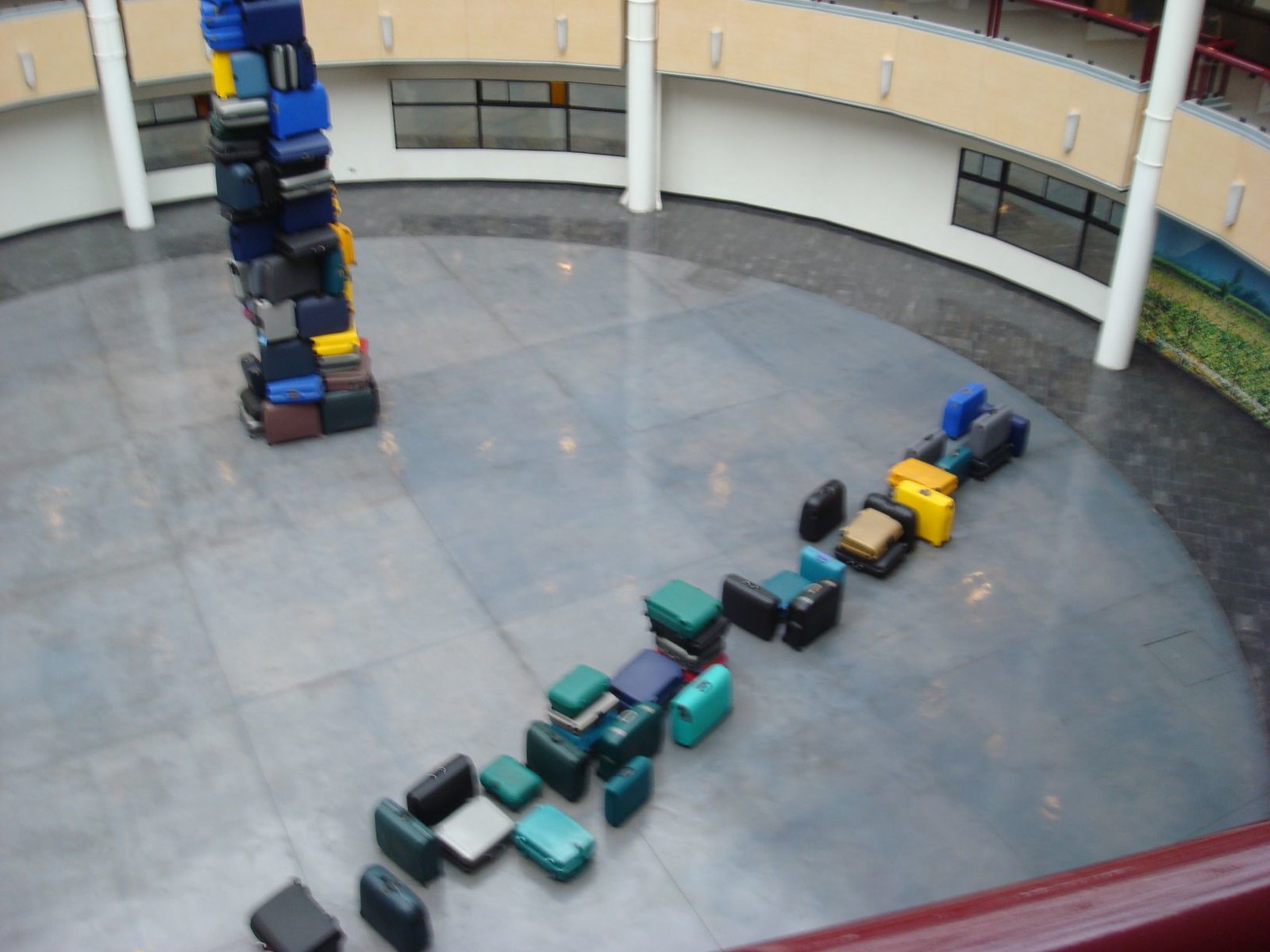The photograph captures a detailed and slightly surreal scene within a large, circular interior courtyard, taken from an elevated vantage point—likely the third or fourth floor—looking downward. The central courtyard features a striking grey, possibly marble floor, with a darker grey circular pattern near its perimeter. The open space is surrounded by white columns and has accents of red railing on multiple levels, hinting at an architectural design that feels institutional, possibly a school or public building.

The ground level showcases two notable arrangements of colorful suitcases. On the left side, there is an impressively tall, totem-like stack of various suitcases, reaching about 20 feet, with colors including blue, yellow, black, brown, and teal. The individual cases in this towering pile are arranged haphazardly, mimicking a game of Tetris or Jenga.

Closer to the middle and stretching towards the bottom left to the upper right, a second row of suitcases lies scattered across the floor. These suitcases are less organized; some are laid flat while others stand vertically, creating an informal line. This row includes colors like green, aqua, black, blue, and yellow, providing a striking contrast against the polished, grey marble floor.

The image, viewed through a slightly blurry window, creates an impression of a cloudy or overcast day and introduces potential motion, adding a dynamic feel to the static display of luggage. The courtyard's serene yet curious atmosphere is accentuated by the careful balance of geometry, color, and the seemingly random yet intentional arrangement of the suitcases.